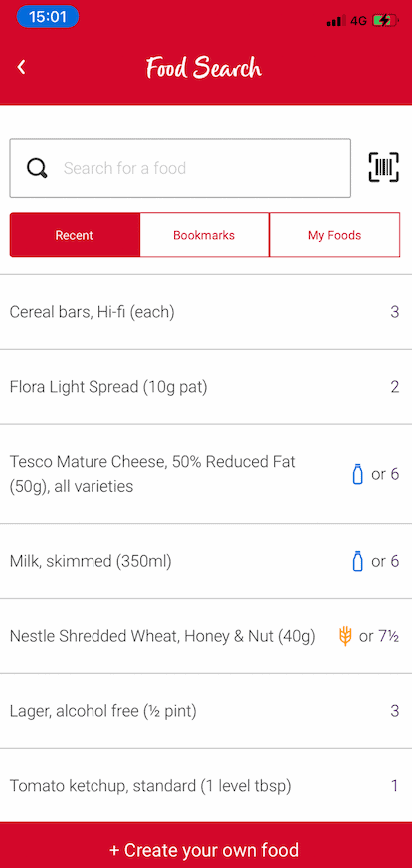This image is a mobile screenshot taken at 15:01 military time, indicated in a blue oval at the top left corner. To the right, there are icons showing full service strength, a 4G connection, and the current battery status.

The primary focus is on a red box labeled "Food Search." Directly below it is a search bar containing the placeholder text "Search for a food," accompanied by a QR code scan button.

The interface is divided into three tabs: "Recent," "Bookmarks," and "My Foods," with the viewer currently on the "Recent" tab. Below these tabs is a list of various food items, each with an associated quantity and a brief description. The measurement units are not explicitly stated but appear to vary by item.

Starting from the top of the list:
1. Cereal Bars, Hi-Fi Each - Quantity: 3
2. Flora Light Spread, 10 grams per pat - Quantity: 2
3. Tesco Mature Cheese, 50% Reduced Fat, 50 grams, all varieties - Quantity: 6 (with a small icon next to it)
4. Milk, Skimmed, 350 milliliters - Quantity: 6 (with a small icon next to it)
5. Nestle Shredded Wheat, Honey and Nut, 40 grams - Quantity: 7.5 (with a wheat icon next to it)
6. Lager, Alcohol Free, Half Pint - Quantity: 3
7. Tomato Ketchup, Standard, One Level Tablespoon - Quantity: 1

At the very bottom of the screen, there is another red box with the text "Create Your Own Food."